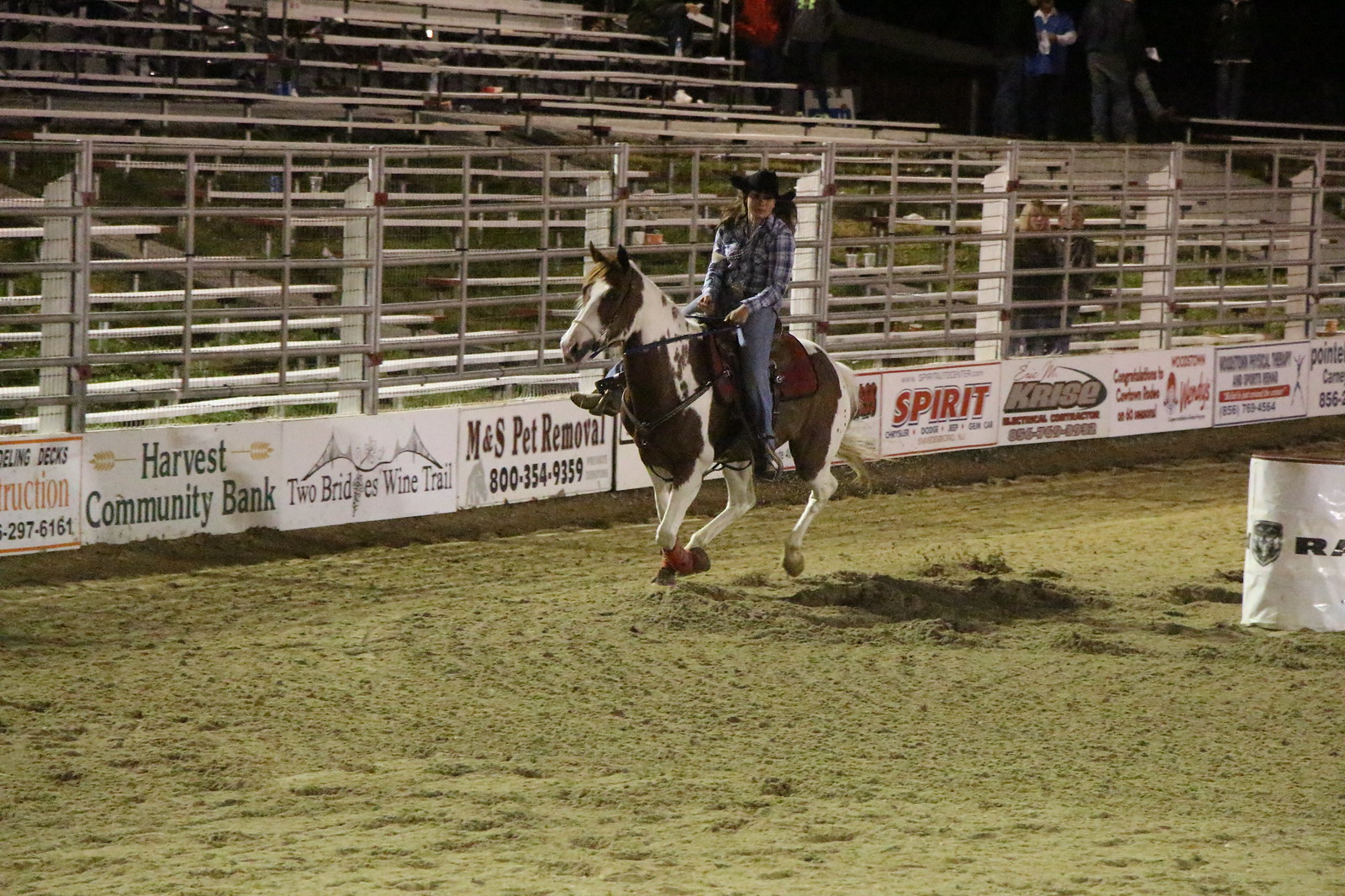In this vivid picture taken at a rodeo event, a young woman clad in flannel and blue jeans demonstrates her skills in a barrels competition while riding a striking brown and white horse. They are captured mid-turn on the dirt, evidence of their hard work and determination. The setting is distinctly rural, featuring numerous sponsor banners along the fence, including names like Dr. M, M&S Pet Removal, Two Birdies Wine Trail, Harvest Community Bank, and KASE. The scene is bathed in quintessential country colors, predominantly white and red. Two spectators are intently watching the action from the front right corner, while the steel bleachers behind them remain largely unoccupied, giving the image a sense of intimacy despite the grandeur of the event.